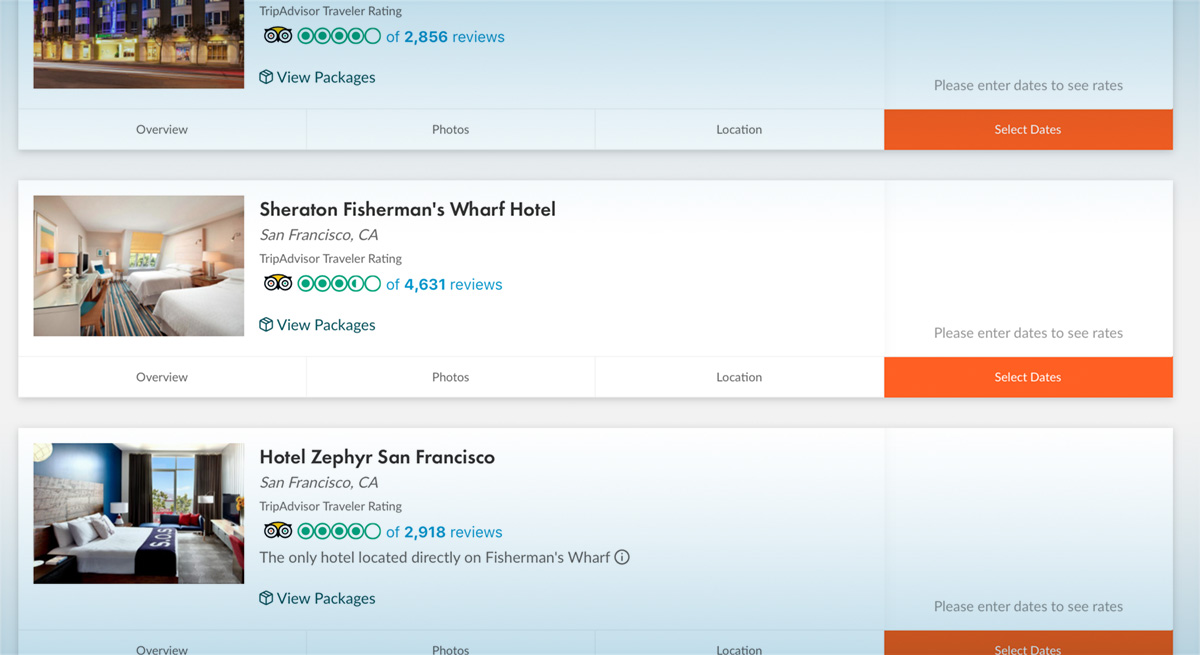Screenshot of a desktop version of a hotel booking site detailing hotels in the San Francisco area. The primary site appears to be TripAdvisor, as indicated by the traveler ratings visible next to hotel names. The two prominently displayed hotels are the Sheraton Fisherman's Wharf Hotel and Hotel Zephyr, San Francisco.

The Sheraton Fisherman's Wharf Hotel is showcased with an image and has received a rating of approximately 3.5 out of 5 stars, based on 4,600 reviews. The rating is visually represented by circles, akin to suns or stars.

Hotel Zephyr, San Francisco, also featured with an image, holds a 4-star rating based on 2,900 reviews. Notably, this hotel claims to be the only one directly located on Fisherman's Wharf, which raises questions since the Sheraton Fisherman's Wharf Hotel carries "Fisherman's Wharf" in its name, hinting at a potential discrepancy.